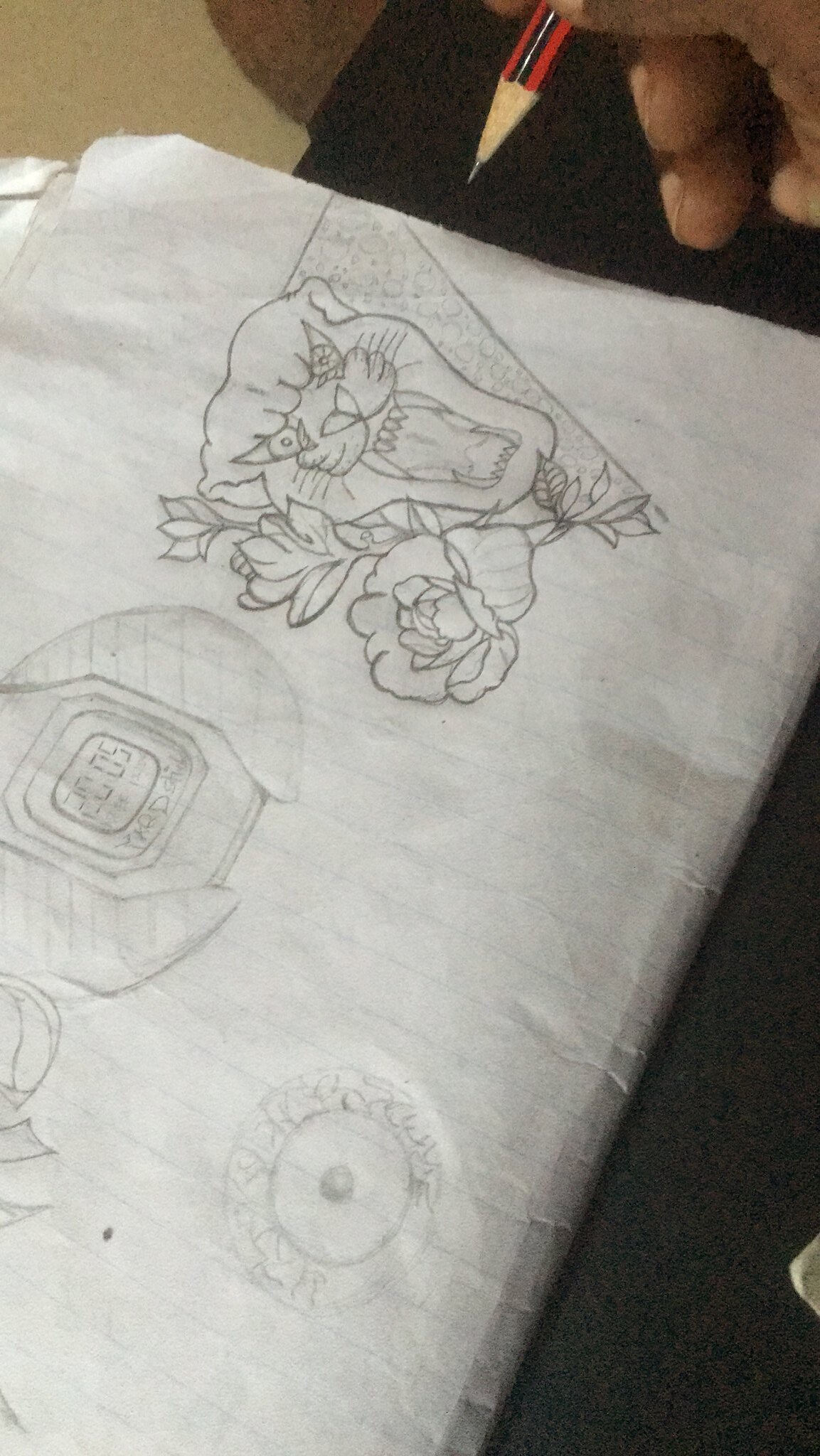A white sheet of paper serves as the background for an eclectic mix of amateur sketches. Thin lines, cages, and balloons fill the backdrop, adding a whimsical element to the collage. At the top of the page, there are delicate drawings of roses. In the center, a bobcat character comes to life with a rough, expressive style. Adjacent to this, a sketch of a growling dog is prominently featured. The bottom left corner displays a detailed drawing of a watch, while a distinct, solitary eyeball illustration is positioned at the bottom, adding an enigmatic touch to the collection.